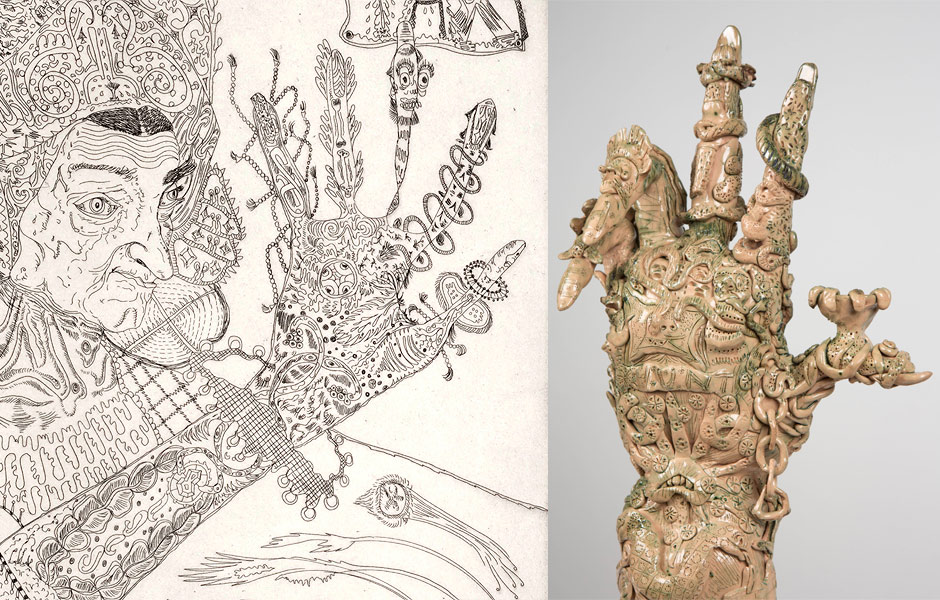This split image displays two artistic representations of the same fantastical hand. On the left, an intricate pen and ink etching portrays a figure with a long nose adorned in elaborate attire, extending a highly detailed, decorated hand. The hand is rich with intricate, fidgety segments, including fingers that transform into various characters and objects: there's a face on the middle finger, other fingers morph into snakes, plants, and even an animated stalk of celery. The hand also features a mesh bracelet and other small detailing in the foreground. On the right side, the drawing is brought to life in a clay sculpture, which mimics the same elaborate patterns and whimsical characters. This sculpted hand, with some fingers bent and others extended, is glazed with patches of light green while retaining the natural tone of the clay. The thumb forms a small bowl, and both hands display consistent decorative themes, emphasizing imaginative details such as faces, chains, and organic elements.